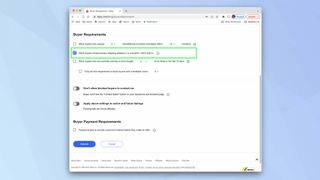The image depicts a low-quality screenshot of a web page, making most of the text illegible and heavily degraded. The primary colors present are green, blue, and white. The screenshot shows a web browser with only one tab open. Due to the poor resolution, the details of the text and any specific information it conveys cannot be discerned.